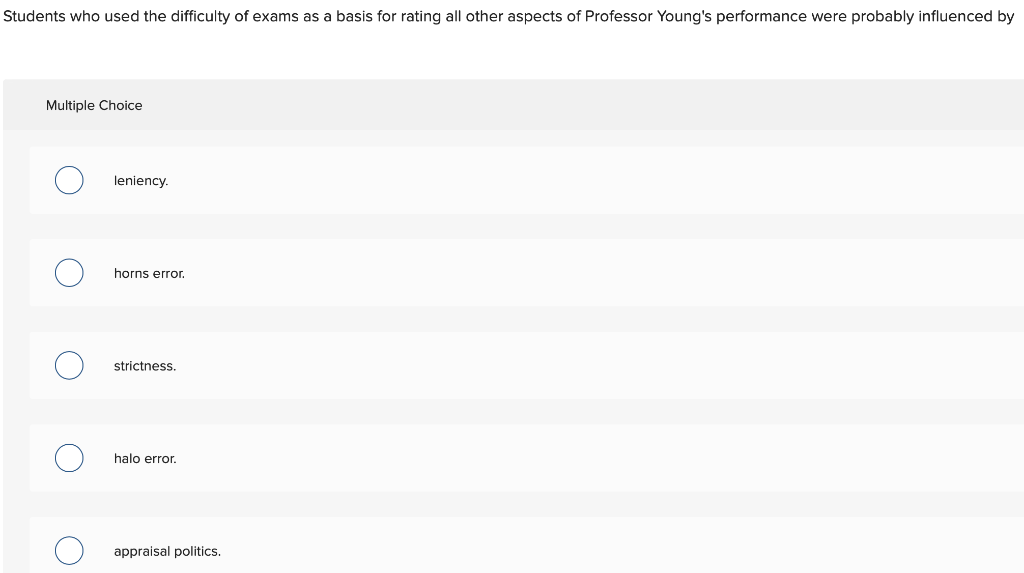The image in question is a simple, straightforward multiple-choice quiz interface. The layout consists of a rectangular frame with a white background at the top against which black text is displayed. The text at the top reads: "Students who used the difficulty of exams as a basis for rating all other aspects of Professor Young's performance were probably influenced by." 

Beneath this question, the background transitions to a lighter gray, which features the words "Multiple Choice" written in black. Below this section, there are five clearly delineated answer options arranged vertically. Each option is paired with a circular selection button, which has a black border and a white interior, indicating that none of the options have been selected yet. Each option is listed in its own section as follows:

1. Leniency
2. Horns Error
3. Strictness
4. Halo Error
5. Appraisal Politics

The image does not contain any additional text, graphics, photos, or drawings. The focus is entirely on the multiple-choice question and its possible answers, presented in a clean and uncluttered format.